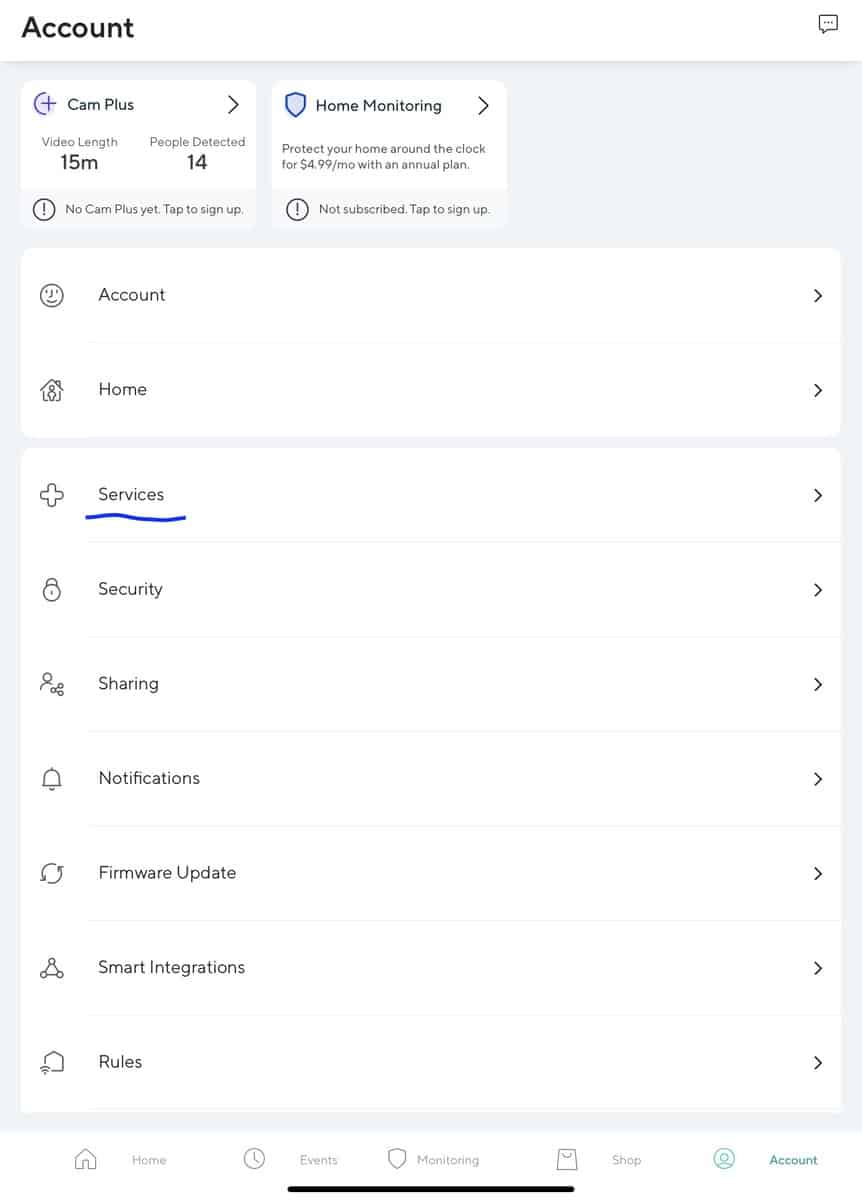In this screenshot, the upper left-hand corner prominently features the word "Account" in bolded black font. On the upper right, a message icon is displayed. The screen has a light blue background with a rectangular shape. In the immediate upper-left section, there are two white rectangles side by side. The left rectangle contains an icon followed by the text "CAM+" and a right-pointing arrow. The right rectangle also has an icon with the text "Home Mentoring" and a right-pointing arrow. Both rectangles have small, unreadable text below them.

Underneath these rectangles, there is a gray circle featuring a small eye icon, followed by very small print. The majority of the remaining screen is organized into horizontal white rectangles separated by thin gray lines, each representing different menu options. On the left side of each rectangle is an icon, followed by the name of the option. On the far right, there is a right-pointing arrow that resembles a lower-case black "v". The list of options from top to bottom includes: Account, Home, and Services—with Services underlined in blue to indicate it is the currently selected option. Following these are Security, Sharing, Notifications, Firmware Update, Smart Integrations, and Rules. The bottom of the screen displays a row of icons that are too small to discern their details.